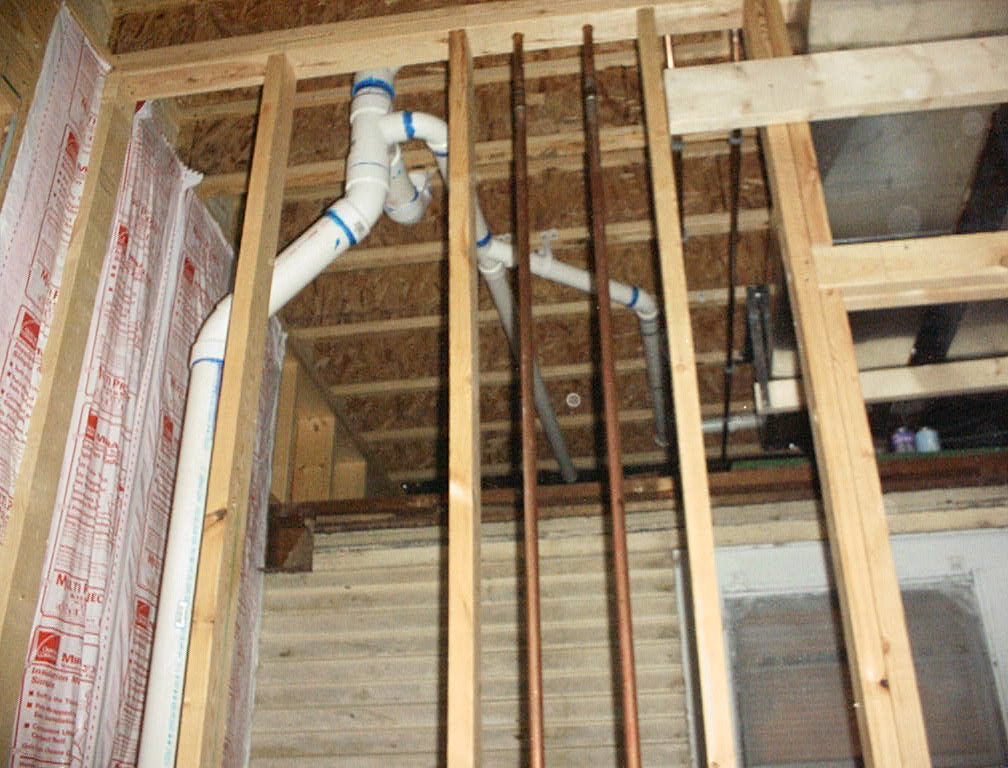The photograph showcases an unfinished section of a house under construction. Prominently featured are exposed wooden 2x4 beams and framing, revealing the skeletal structure of the building. White PVC pipes, likely part of the plumbing, run vertically from the ceiling and horizontally underneath the floor of the room above. These pipes feature turquoise-blue markings, possibly tape, indicating connection points or areas of interest. Copper pipes also weave through the structure, contributing to the plumbing system. On the left side of the image, white and red plastic sheeting, possibly insulation packaging, is visible. The ceiling appears to be made of a brownish-beige material that resembles cork. The wooden beams vary in color from light beige to richer brown hues, adding texture to the unfinished space. Overall, the image captures the raw, in-progress state of the house's construction, focusing on the essential building materials and plumbing installations.